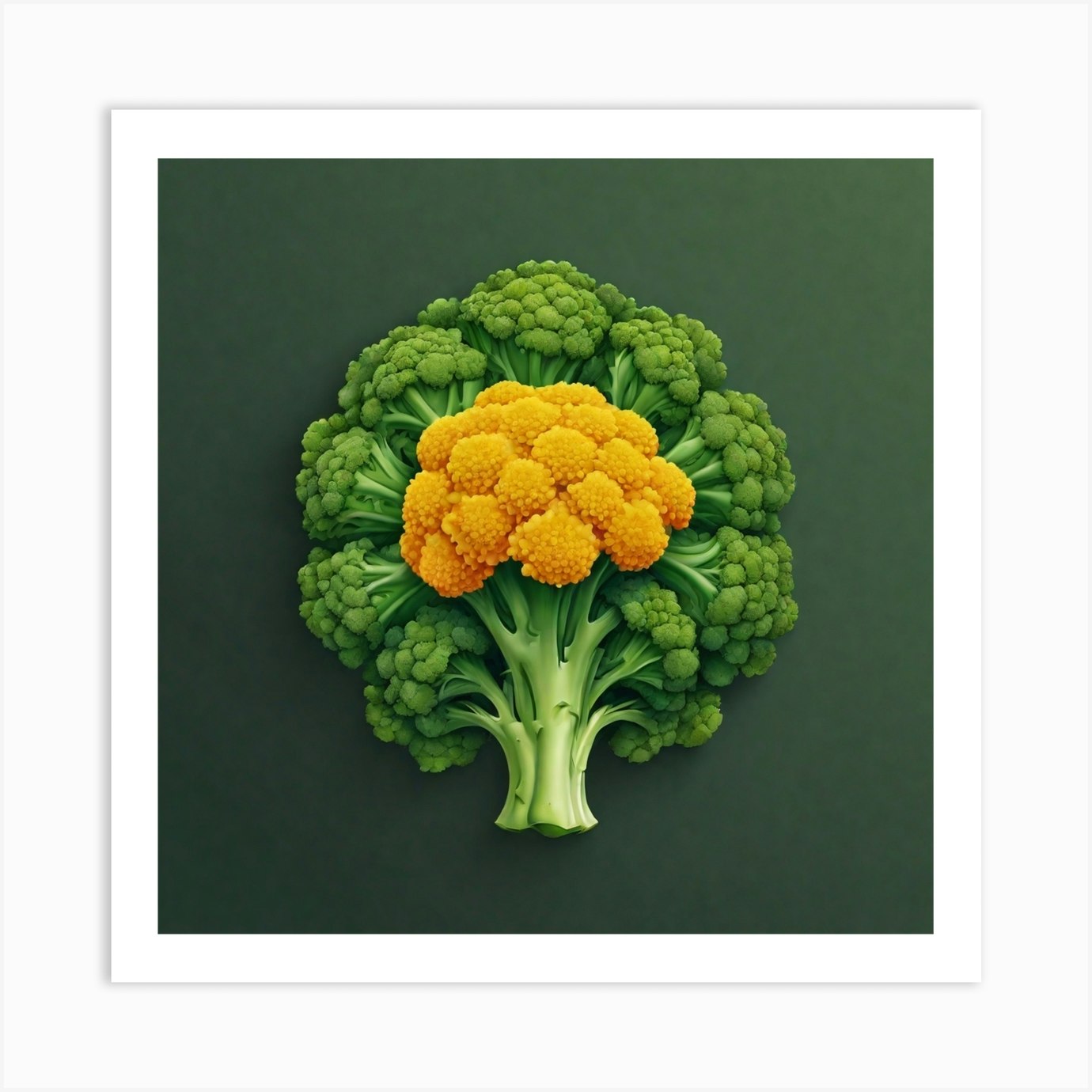This 3D style illustration, highly rendered and square in shape, showcases a surreal and highly detailed depiction of broccoli against a deep forest green background. In the center of the composition is a dominant, large clove of broccoli with smaller clusters branching off. Intriguingly, one of these clusters is an unnatural goldish-yellow color, creating a visually striking contrast. The abstract, AI-generated artwork features smooth, curved lines, lending an otherworldly, almost unsettling quality to the broccoli's form. The image is encased in a white border, giving it the appearance of a digital print with a drop shadow effect, further emphasizing its artificial nature.